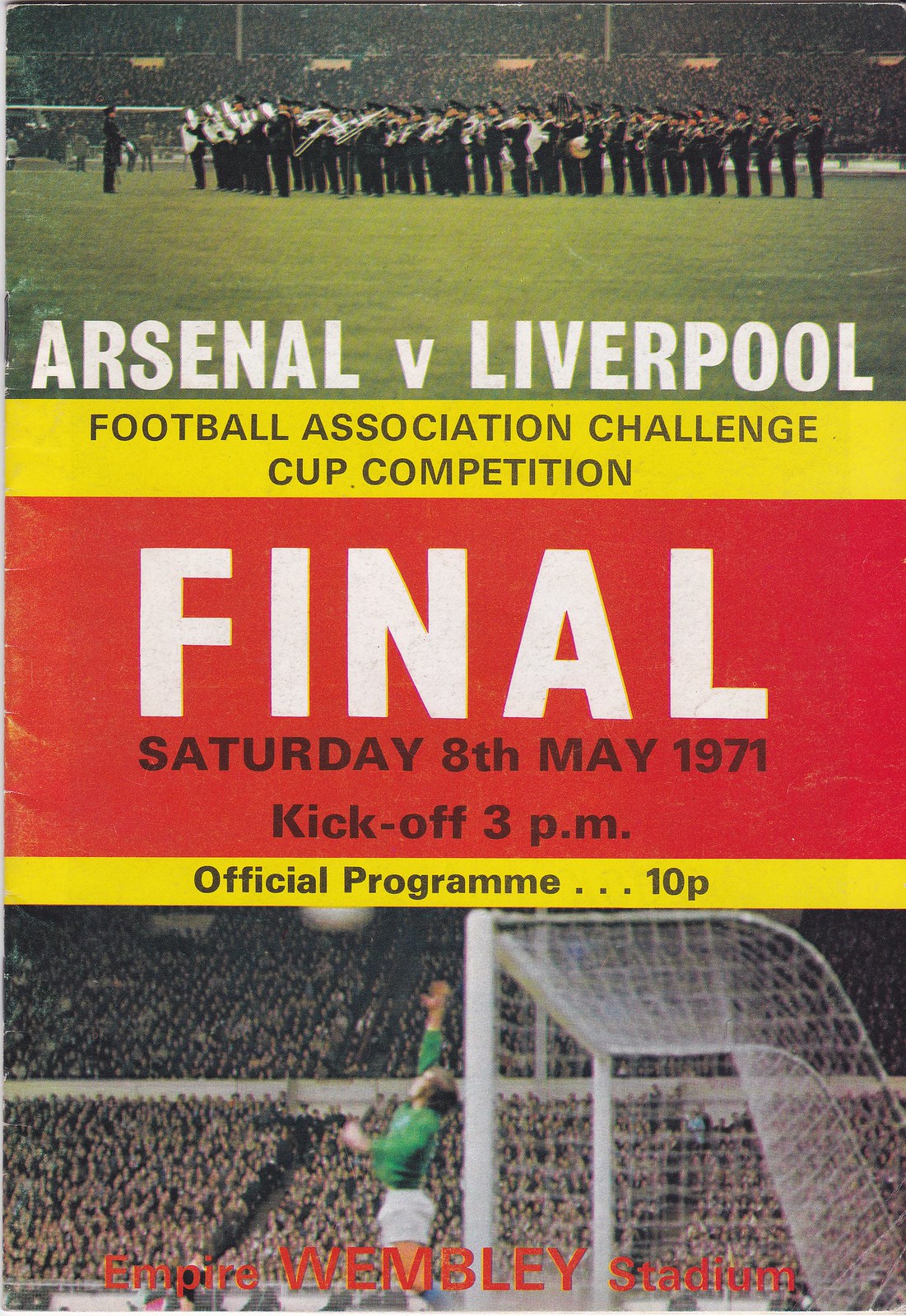This image is an advertisement for the Football Association Challenge Cup Final held on Saturday, May 8th, 1971. The advertisement is divided into three sections. At the top, a vibrant image shows a marching band performing on a packed football field, with the stands filled to maximum capacity. Above this scene, in bold white text, it reads "Arsenal vs Liverpool.” The middle section provides detailed information about the event, stating: "Football Association Challenge Cup Competition," followed by "Final" in large white letters. Below this, it gives the date and time: "Saturday, 8th May, 1971, kickoff, 3 p.m." It also mentions the official program price as "10-P." The bottom section features a dynamic side-view photograph of a goalie leaping to block a soccer ball aiming for the goal. This intense moment is juxtaposed with the inscription "Empire Wembley Stadium" in red text, prominently placed at the bottom.